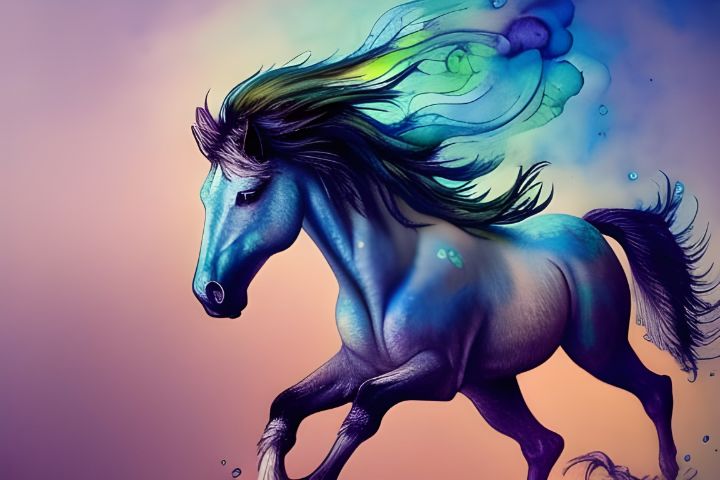The image is a vivid, digital fantasy painting featuring a horse in a full gallop, captured with extraordinary detail and imaginative color schemes. The horse, positioned prominently and running towards and slightly past the viewer, has an iridescent blue body that transitions to a deep purple on the legs and lower stomach. This iridescence, combined with purples and pinks, gives the horse an almost glowing, luminescent appearance.

The mane and tail of the horse are particularly captivating, as they billow dramatically in the breeze. The mane, predominantly blue, shifts into shades of green and yellow, creating a psychedelic liquid pattern that appears to be dripping multicolored dyes and paints in the air behind it. The tail echoes this effect, leaving droplets suspended in mid-air.

The background of the image features a striking color gradient, transitioning from a glowing peach-orange at the center to rich purples in the corners. This background is adorned with little splotches of blue and greens that float around, enhancing the fantastical atmosphere of the scene. Overall, the image is a mesmerizing work of art that leverages an array of imaginative colors and digital techniques to create a truly otherworldly depiction of a galloping horse.